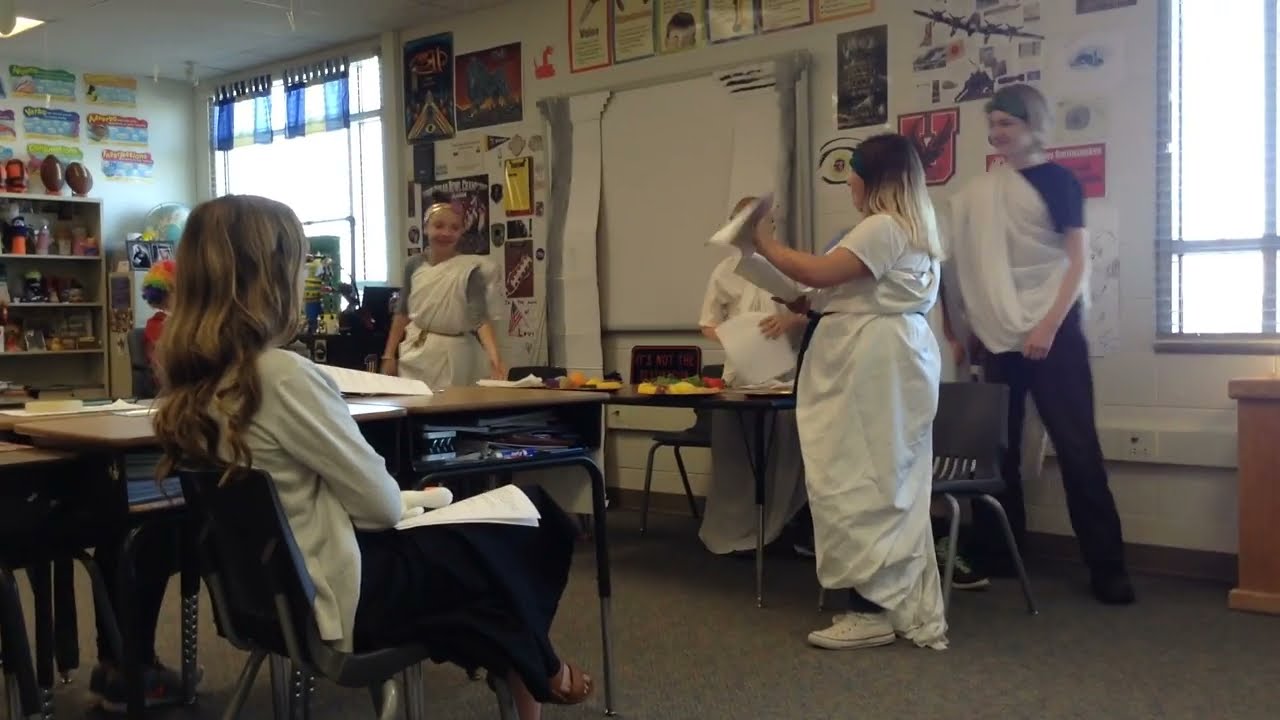The image depicts a bright and vividly decorated classroom where a blonde teacher, dressed in a white shawl and black skirt with brown sandal shoes, is seated on the left side in a student’s chair at their desk, holding a stack of white papers in her lap. She is observing a group of five students who are dressed in togas, suggesting they are rehearsing or performing a play. The scene is filled with energy as the four students on the right, who are smiling, are looking towards the fifth student on the left. The classroom walls are adorned with an array of papers, art, and decorations, creating a vibrant and stimulating environment. Prominently, there are two big windows letting in bright daylight, making the room feel expansive and airy. Centrally placed is a whiteboard, while a shelf on the far left displays various objects, including two noticeable footballs. The floor is carpeted, adding to the cozy atmosphere. The desks in the foreground, possibly part of the play’s set, have some fruits placed on them, adding to the scene’s theatrical setting.